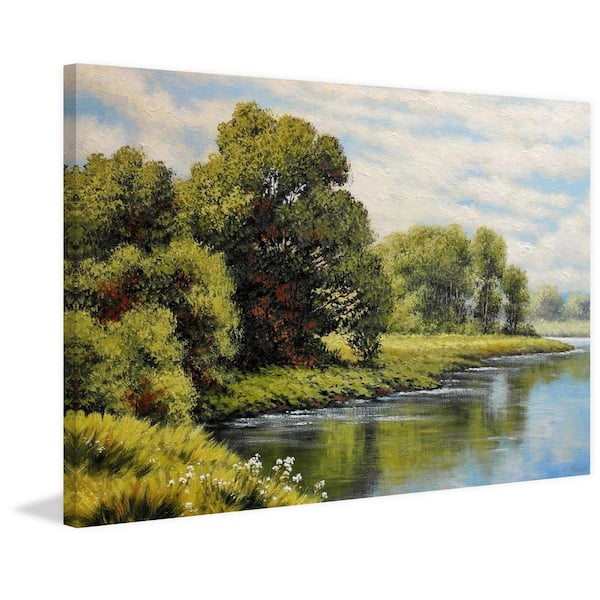The painting, an oil piece on a thick, framed-less canvas, depicts a serene lakeside landscape under a partly cloudy, blue sky. Large green trees with varied shades—from vibrant green to deep browns and blacks representing the shadows—line the grassy bank of the calm lake. The stillness of the water beautifully mirrors these trees and the sky above, enhancing the painting's tranquil atmosphere. Foreground details include yellow-green grasses and delicate white wildflowers, leading the viewer's eye to the reflective, tranquil water. The background extends to more tree-covered areas, all blending harmoniously into the lush, green landscape. The texture of the paint adds depth, particularly visible in the sky and the rippling effect along the water's edge. This idyllic and serene lakeside scene, reminiscent of Bob Ross's peaceful landscapes, is photographed against a stark white backdrop with a slight drop shadow at its bottom left corner, emphasizing its three-dimensional quality.